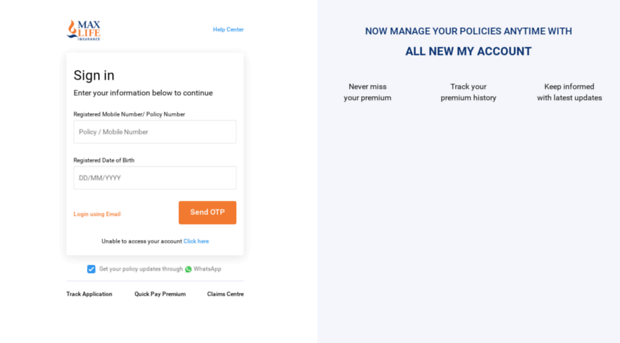Against a stark white background, a small square measuring approximately 1.5 inches on each side commands attention. Its outline is delicately traced in gray. The upper right corner of the square appears to fold inward, forming a downward-pointing triangle cutout. Inside the square, the scene is subtly detailed: the upper region features a light blue background with a tiny, white squiggly line, suggestive of a drifting cloud. Below the cloud, a patch of green evokes the image of a serene hill or mountain. To the right of this green area, a diagonal white line cuts through the space, adding an element of simplicity and intrigue. This minimalistic image is confined entirely within its small, 1.5-inch boundary, presenting a concise yet evocative visual narrative.